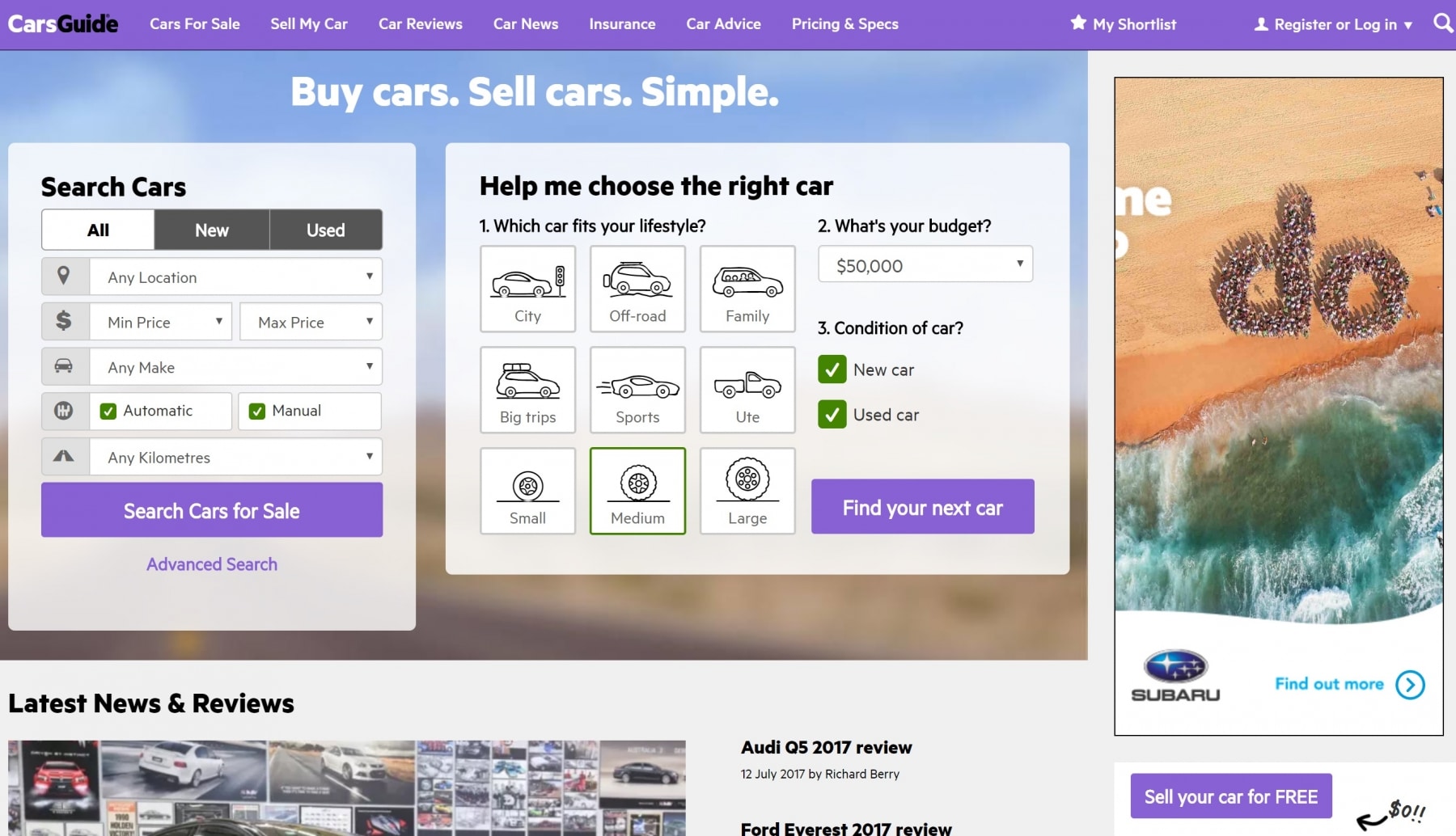The screenshot depicts the homepage of the Cars Guide website, predominantly featuring a light purple accent color. At the top of the page, there is a header menu with a white and black "Cars Guide" logo on a purple background. The menu includes options labeled as "Cars for Sale," "Sell My Car," "Car Reviews," "Car News," "Insurance," "Car Advice," and "Pricing and Specs."

On the top-right side of the header, there are additional icons and options: a star icon labeled "My Shortlist," a head-and-shoulders icon for "Register or Log In," and a magnifying glass for search functionality. All these elements are displayed in white on the same purple background.

On the right side, there's an advertisement for Subaru featuring an image of a wave crashing onto sand with the words "Subaru" and "Find out more." Below this ad, there is a prominent button labeled "Sell your car for free" with an arrow and "0$!!"

The main section of the page features a blurred background image of a road flanked by desert scenery under a beautiful blue sky, overlaid with the bold text "Buy cars, sell cars simple." Beneath this header, there is a car search section with various drop-down boxes for "All, New, or Used" cars, location, minimum price, maximum price, car make, transmission type (automatic or manual), and mileage options. Users can click a purple button labeled "Search cars for sale," or access an "Advanced search" link also in purple.

Additionally, there is a "Help me choose the right car" section with three key questions:
1. "Which car fits your lifestyle?" offering nine buttons such as City, Off-road, Family, Big Trips, Sports, Utility (a truck icon), and size options Small, Medium, and Large.
2. "What's your budget?" with a drop-down menu showing a default value of 50,000.
3. "Condition of car" displaying checkboxes for New and Used cars, both of which are currently selected. Below this section is another button labeled "Find your next car."

At the bottom of the page, there is a section for "Latest news and reviews," featuring numerous pictures and links to related articles.